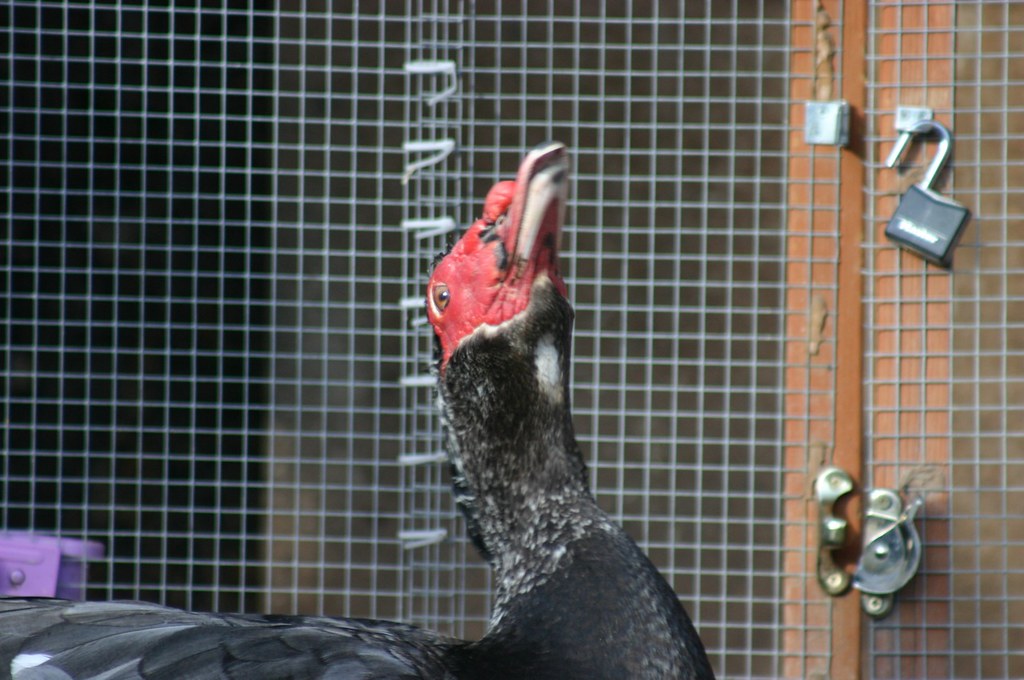The photograph captures a black-feathered bird, likely a turkey or possibly a turkey vulture, inside a cage. The bird has a striking red head that is prominently covered in fleshy, textured skin typical of turkeys. Its beak is a mix of red and white hues and is rounded, somewhat resembling the beak of a duck. The bird's head is tilted sharply backward, as if in mid-squawk, with its beak closed and one eye visible, giving a clear side profile from its shoulders up. In the background, the cage is visible with vertical and horizontal thin metal wires, and a wooden frame. There is an unlocked padlock on the cage door and a rotating bolt lock underneath it, both made of metal. Only the upper half of the bird is visible, from just above its wings to its head.